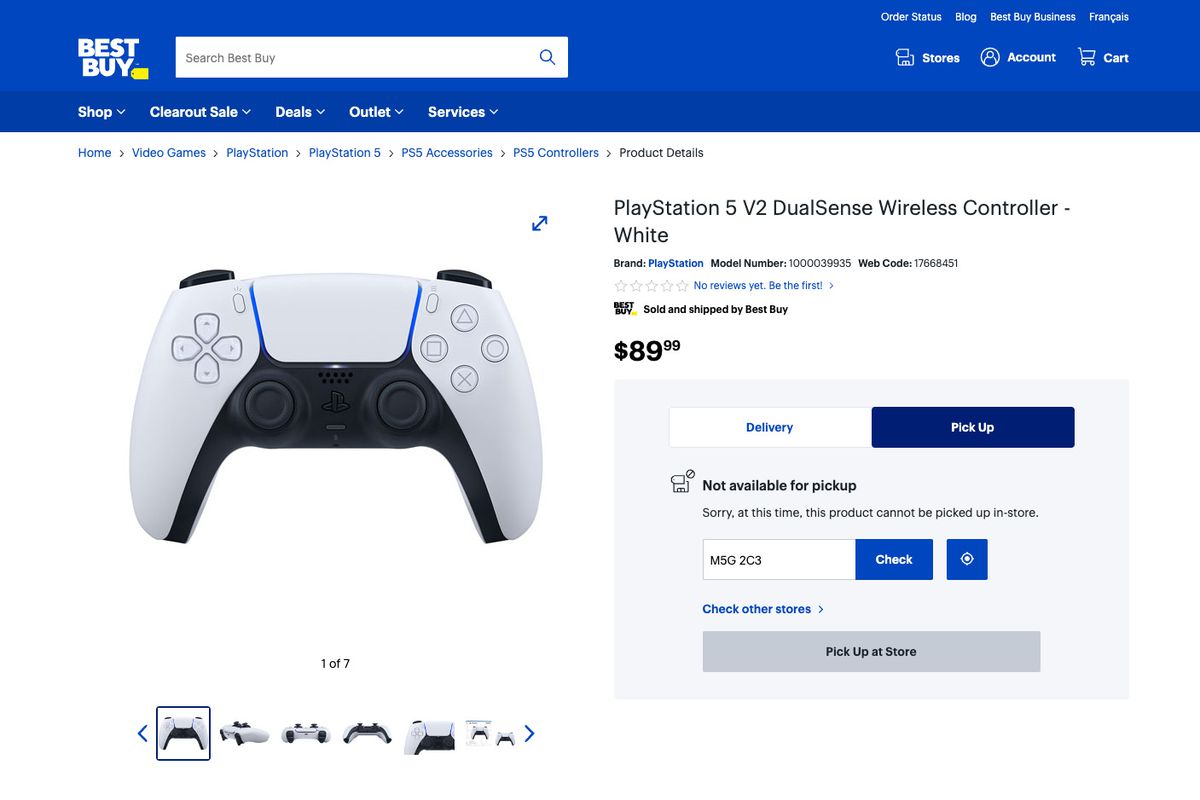The Best Buy website page displays a clean and organized layout. In the upper left corner, the "Best Buy" logo is prominently featured. Adjacent to the logo is a search bar with an accompanying magnifying glass icon. To the right of the search bar, there are several links: 'order status,' 'blog,' 'Best Buy France (Presnus, France),' 'stores,' 'account,' and 'cart.'

The highlighted product is a "PlayStation 5 V2 DualSense Wireless Controller" in white. The product details are as follows: 
- Brand: PlayStation
- Model Number: 1004039935
- Web Code: 17668451
The product has no reviews yet, encouraging customers with a "Be the first to review" message in blue text. 

The controller is sold and shipped by Best Buy, priced at $89.99. Two buttons are available for purchase options: 'Delivery' (displayed on a white button with blue text) and 'Pickup' (displayed on a blue button with white text). However, the item is currently not available for in-store pickup, as indicated by the message below the purchase options.

There is a text field labeled "M5G2C3" next to a blue 'Check' button in white font, suggesting an option to check availability by location. Further below, there is a 'Pick up at other stores' option presented as a gray button along with another option to check availability at other stores.

An image of the PlayStation 5 DualSense Controller is featured prominently, showing off its sleek design with a predominantly white color accented with black and blue details.